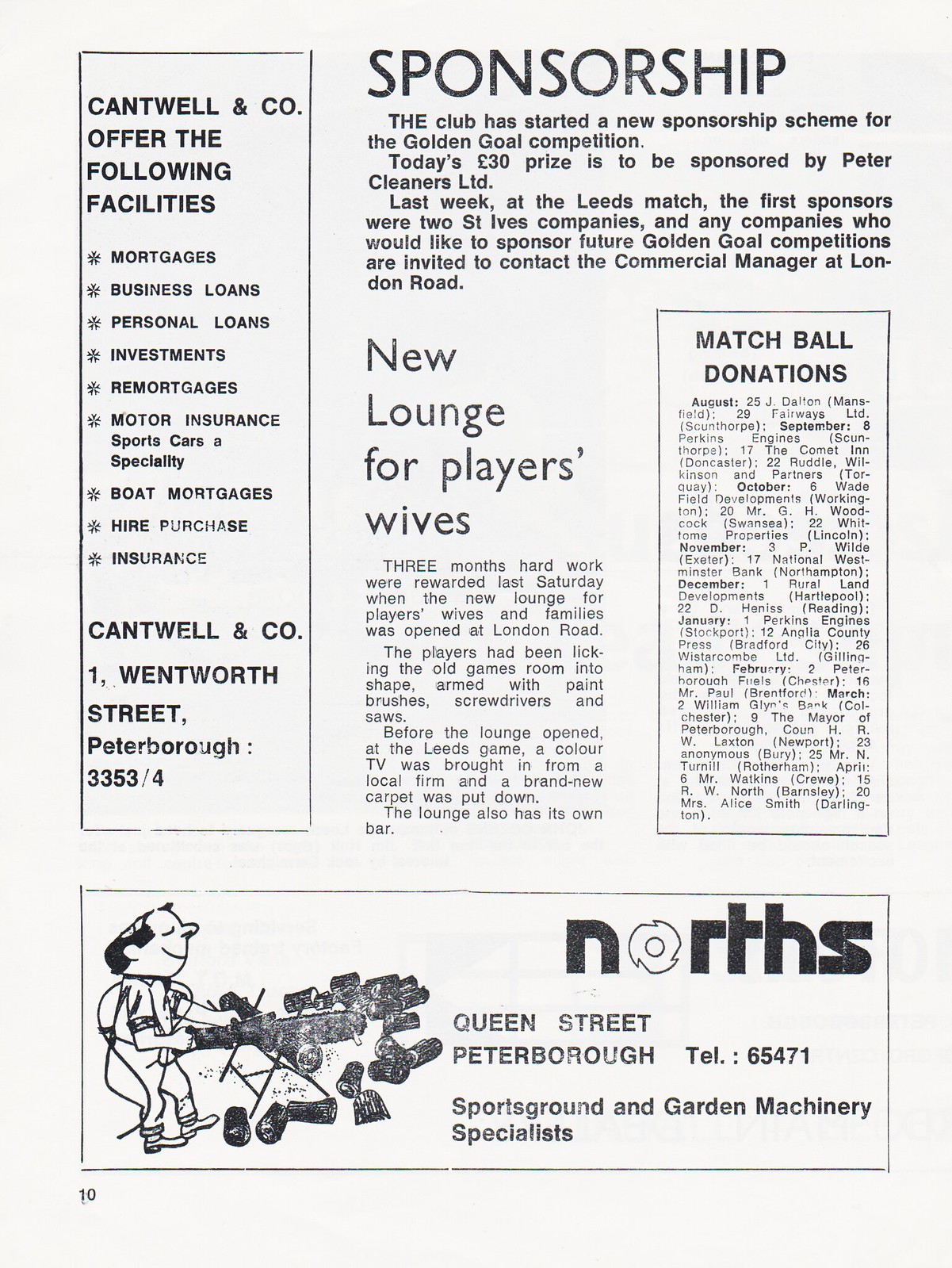This page, seemingly from an aging magazine, serves as a newsletter for a sports team, detailing recent sponsorship and club developments. At the top right, the header "Sponsorship" introduces the club's new sponsorship scheme for the Golden Goal competition, with Peter Cleaners Limited sponsoring today's €30 prize. Last week's prize at the Leeds match saw sponsorship from two St. Ives companies. The club invites future sponsors to contact the commercial manager at London Road.

Beneath this, a section titled "New Lounge for Players' Wives" celebrates the unveiling of a new lounge for players' families, located at London Road. Prepared with significant effort over three months, the lounge boasts a color TV contributed by a local firm, a new carpet, and its own bar. The players helped prepare the game room using paintbrushes, screwdrivers, and saws, completing the lounge just before the Leeds game.

On the left side of the page, Cantwell & Co. advertises their services, which include mortgages, business and personal loans, investments, remortgages, motor and boat insurance, and hire purchase insurance. Their contact details are listed as 1 Wentworth Street, Peterborough.

Towards the right, "Match Ball Donations" appears in a large boxed section, while an illustration at the bottom shows a man using a chainsaw to cut logs north of Queen Street, Peterborough, accompanied by contact details for a local sports garden machinery specialist. The page is marked with "Page 10" and exudes the character of a well-worn magazine.